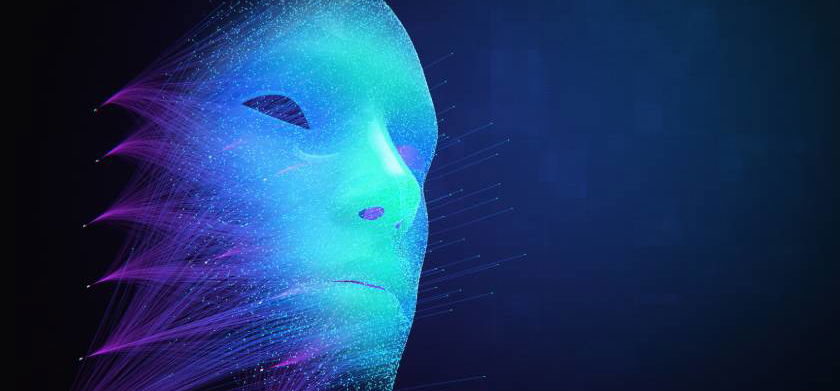The nighttime photograph showcases an intricate outdoor art installation, featuring a mask seemingly assembled from thousands of tiny white laser lights. Set against a dark blue-black sky, the mask, which appears gender-neutral, is formed by vertical strings of lights meticulously arranged to create a cohesive face. On the left side of the mask, five bright light points serve as the origin from which vibrant lines radiate, initially purple before transitioning through light blue to white, weaving together to portray facial features such as the right eye, nose, and mouth. The striking contrast between the luminous mask and the surrounding darkness highlights the ethereal and techno-like aesthetic of the installation.